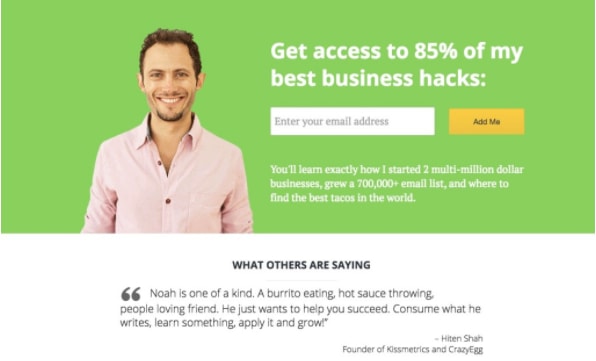In this horizontal, rectangular image, we see part of a website featuring a section for users to enter their email address and leave a comment or review below. The top part of the image has a green background. On the left side, there is a front-facing view of a person, shown from the upper torso up, with a light skin tone, short black hair, and a warm smile that reveals their top row of teeth. They are wearing a pink dress shirt.

To the right of the person, the text reads, "Get access to 85% of my best business hacks." Below that, there is an option to enter an email address followed by a button labeled "Add Me," which is an orangish rectangle with black text. Further down, the text explains, "You'll learn exactly how I started two multi-million dollar businesses, grew a $700,000+ email list, and where to find the best tacos in the world."

The bottom half of the image has a white background. It includes a testimonial section titled "What others are saying," which features a quote: "Noah's one-of-a-kind, a burrito-eating, hot sauce-throwing people-loving front. He just wants to help you succeed. Consume what he writes, learn something, apply it, and grow." This testimonial is attributed to Hiten Shah, the founder of Kissmetrics and Crazy Egg.